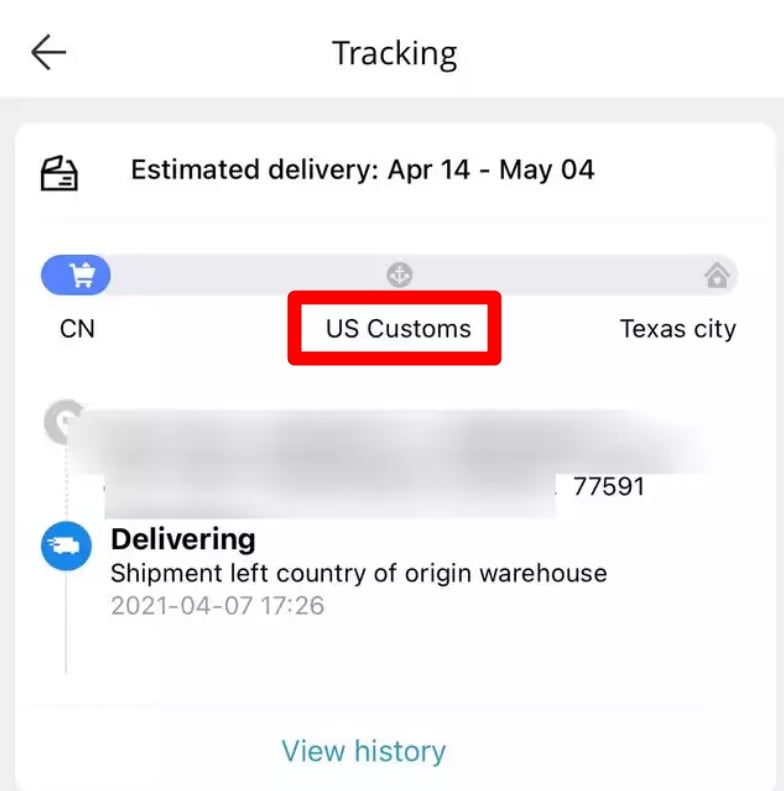This image is a detailed screenshot of a phone screen displaying a package tracking interface for an international shipment. At the top center of the screen, the word "Tracking" is prominently displayed, signaling the function of the page. In the top left corner, a back arrow icon is visible for navigating back to the previous screen.

Directly below this is a gray-bordered box with a white background. On the top left within this box, there is a black and white package icon. Adjacent to the icon, the estimated delivery dates are provided, stating "Estimated Delivery April 14th to May 4th."

Underneath the estimated delivery information, there is a progress bar that indicates the shipment's status. The progress bar is partially filled with blue, suggesting the package's journey. The leftmost section of the progress bar displays a shopping cart icon, while the middle features an anchor-like icon. On the far right end of the progress bar, there is a home icon. The blue fill extends just past the shopping cart icon, indicating initial shipment progress. Below this blue-filled section, the label "CN" is visible, likely representing the country of origin, China.

The anchor icon in the middle is labeled "U.S. Customs," enclosed in a red box, highlighting its significance in the shipment process. To the right, below the home icon, "Texas City" is listed as the final destination.

Further down, there is address information displayed, but it is blurred for privacy, with only the zip code "77591" legible. At the bottom of the box, it states, "Delivering. Shipment left country of origin warehouse on 2021-47 at 07:26." Below this, a "View History" link is provided for more detailed tracking history.